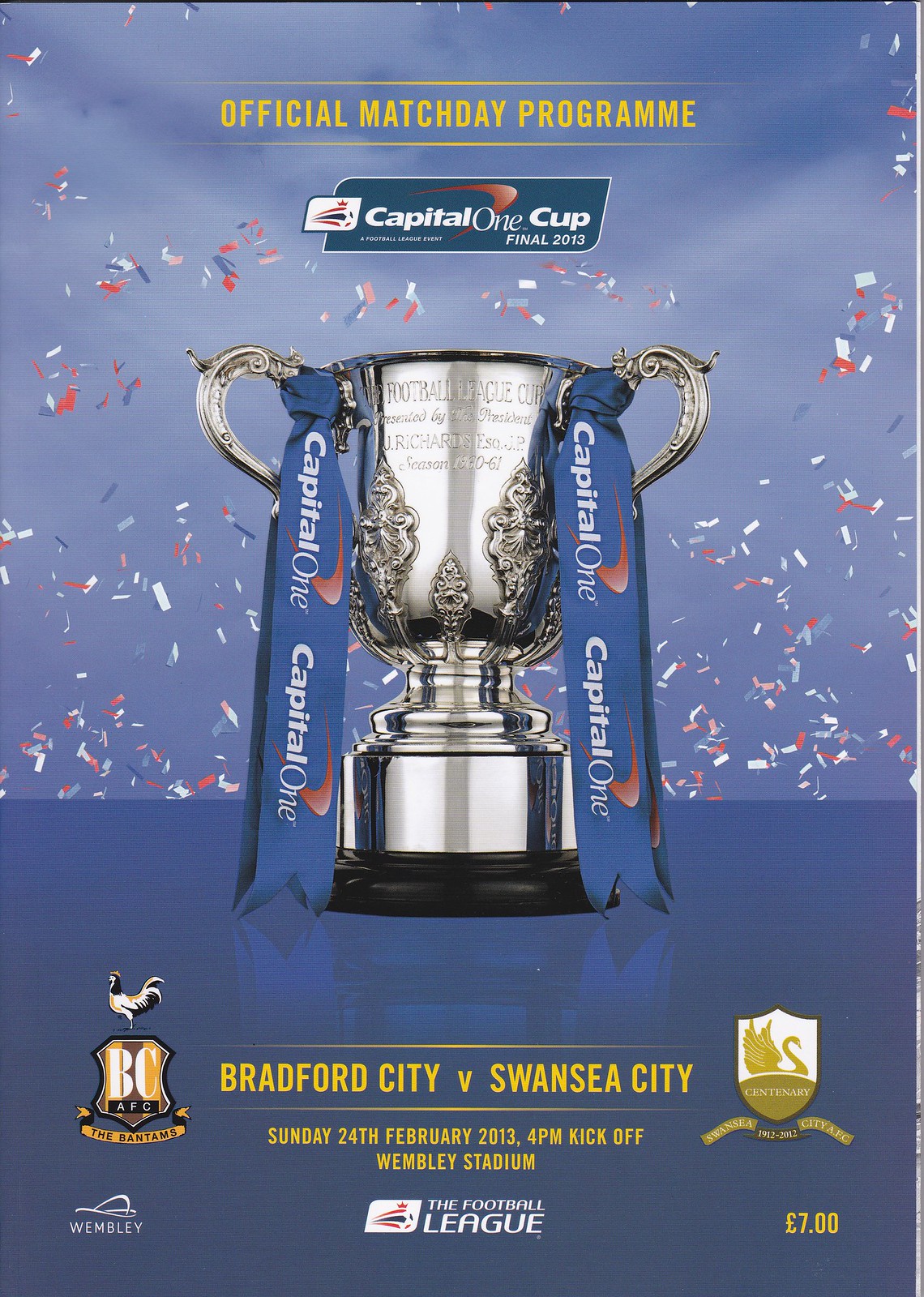The poster features a light blue background that fades into white. At the top, in bold yellow capital letters, it reads "OFFICIAL MATCH DAY PROGRAM." Below this is a green banner with the Capital One Cup logo, featuring a red boomerang shape with white text that reads "Capital One Cup Final 2013." Central to the design is a silver trophy adorned with blue and red Capital One ribbons hanging from each handle. Surrounding the trophy are light blue, white, and orange confetti. The text below the trophy, also in yellow, announces "Bradford v. Swansea City, Sunday, February 24, 2013, 4 p.m. kickoff, Wembley Stadium." Further down, in white, it says "The Football League," flanked by two crests: one bearing a chicken and BC on the left, and the other a swan on the right. At the bottom left is a Wembley logo in white, and on the bottom right, in gold, it states "Seven Pounds."